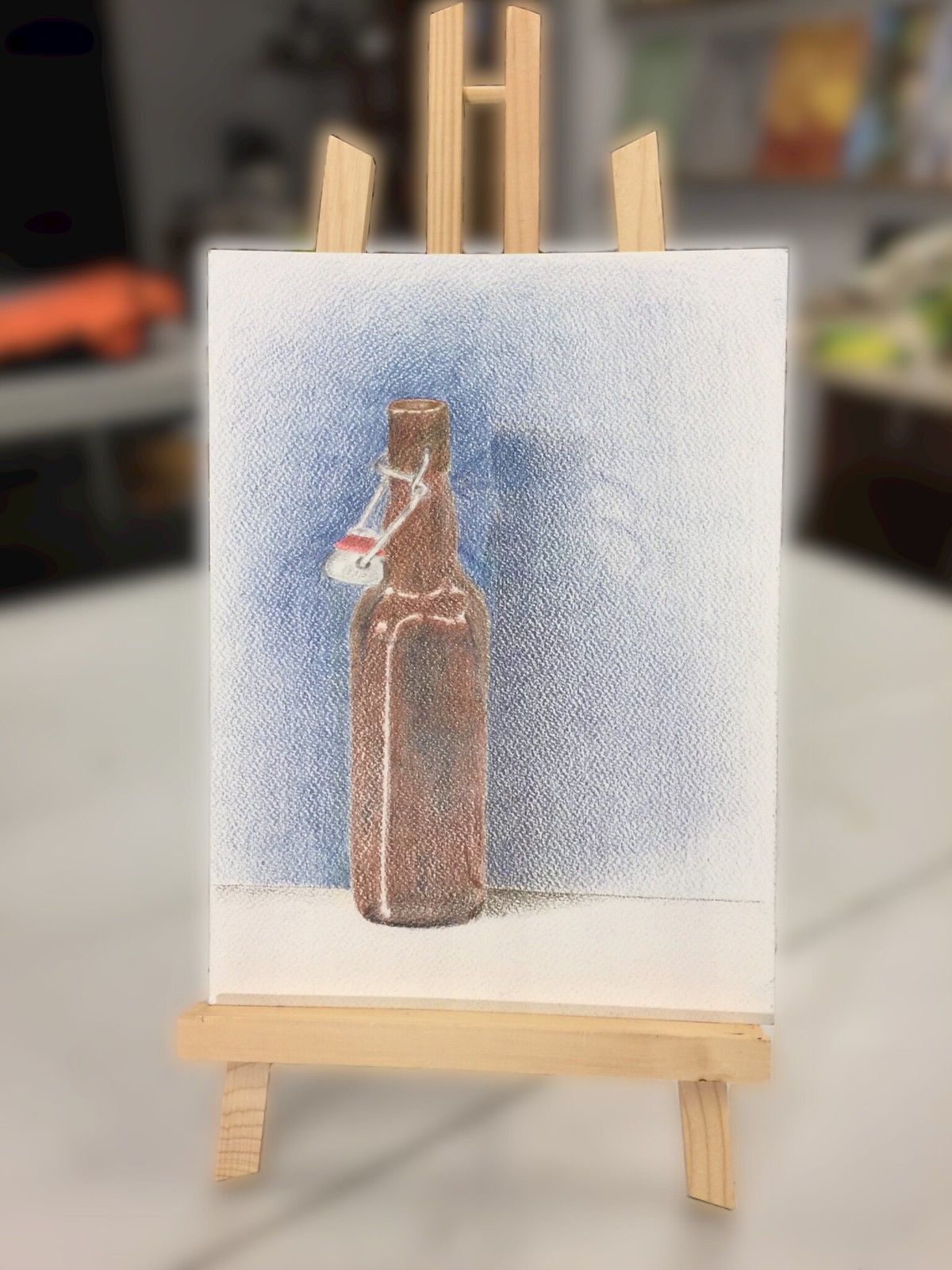In the image, we see a highly detailed photograph of a small piece of art displayed on a wooden easel with a natural finish. The easel sits on a white surface, possibly a tabletop or countertop. The background behind the easel is intentionally blurred, making it difficult to distinguish whether it's a kitchen with countertops or a shop with a sales counter, thus drawing full attention to the artwork itself.

The artwork, possibly a painting or a pastel drawing, depicts a brown amber bottle with a wire bale and a white ceramic stopper, the top of which is open and hanging off to the left side. The bottle features white highlights and is set against a background that transitions from a purplish-blue hue near the center to white around the edges. The bottle stands on a white flat surface within the artwork, casting a visible shadow on a blue-shaded wall behind it. The image includes no text, keeping the focus solely on the artistic elements presented.